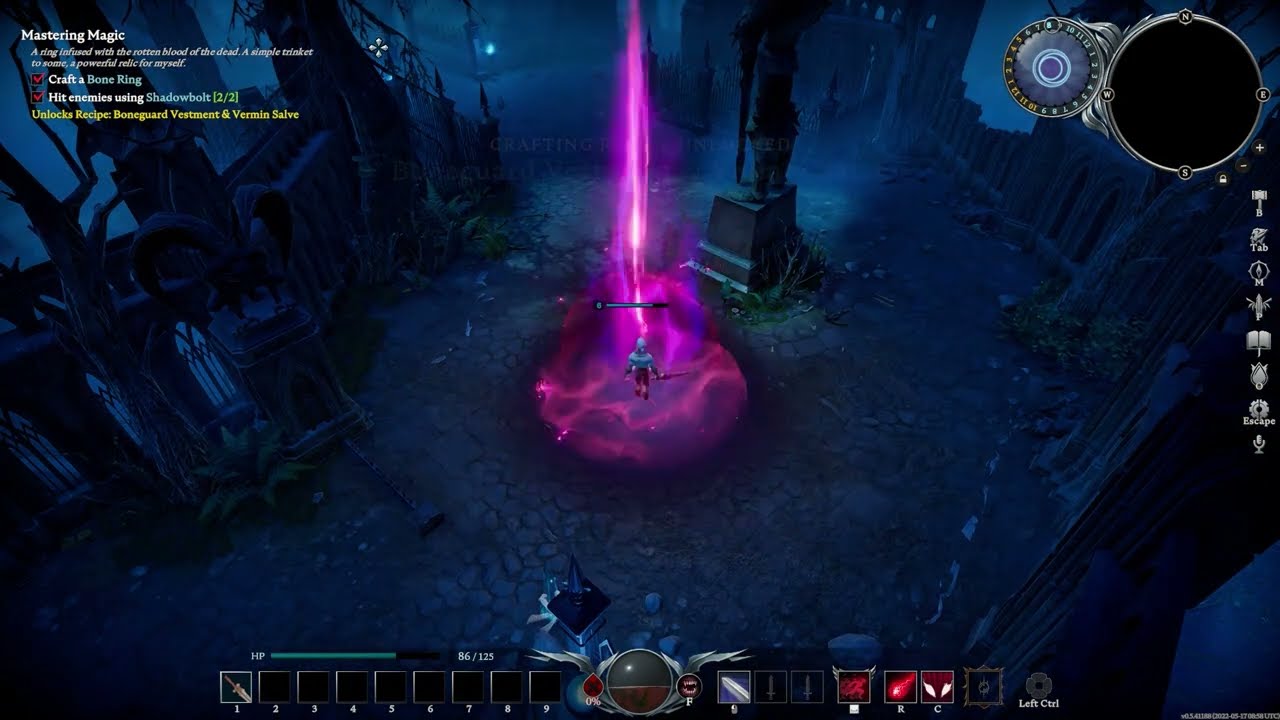The image depicts a dark, atmospheric scene from a video game, possibly set in a dimly lit alley at night. Dominating the center is a radiant, neon pink and purple cone-shaped structure, emitting a bright white light beam from its core. Lightning-like arcs in purple energize the scene, giving it a dynamic, electric feel. At the base of this luminescent structure stands a game avatar, depicted as a green and red figure wielding a sword in their left hand, enveloped in a cosmic cloud-like effect, suggesting either a dramatic landing or launching animation.

In the upper left corner of the image, there are six rows of small, white and yellow text, too detailed to discern individually but evidently crucial for the gameplay or storyline. The upper right corner features a duo of concentric circles; the outer one is black with silver encrusting and cardinal directions marked, while the inner one is a grayish gear or progress indicator. Additional circles are visible on the periphery, signifying various game metrics or statuses.

Icons line the right edge, organized vertically, likely representing tools, scores, or other game functions, with a count of seven in total. Along the bottom of the image is a horizontal bar containing a series of square panels—ten on the left, followed by a central gray sphere with a light gray design, and eight more white-outlined squares extending to the right. This layout is typical of a gaming interface, providing players with essential controls and information at a glance.